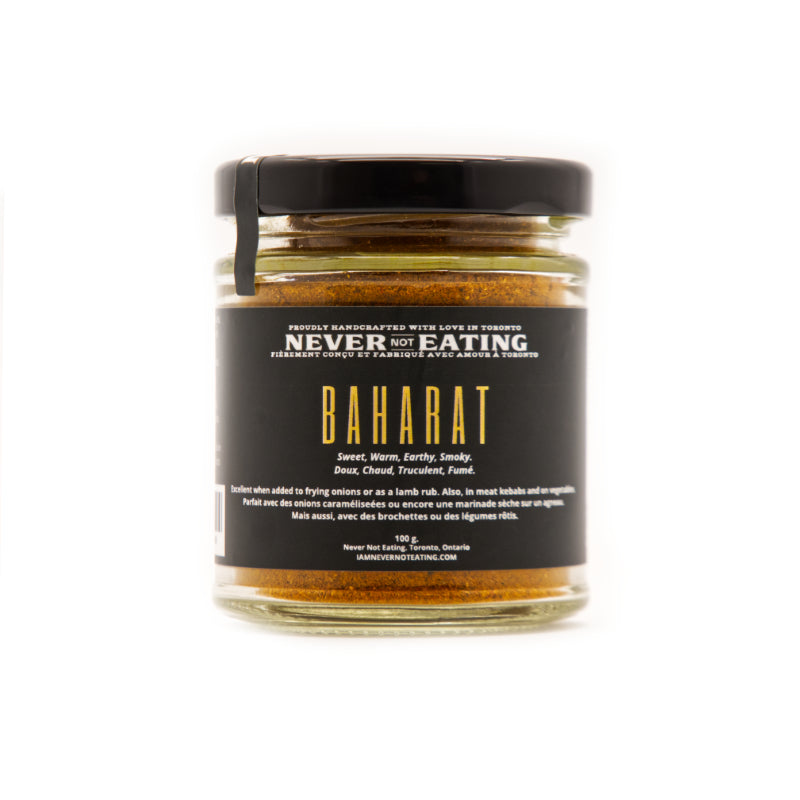This detailed photograph showcases a clear glass jar filled with a reddish-brown seasoning, prominently set against a stark white background, providing a minimalistic yet sharply focused view often seen on retail websites. The jar features a black metal lid secured with a small seal to ensure it hasn't been tampered with. Wrapped around the jar is a sleek black label adorned with various inscriptions.

At the top of the label, in white letters, it proudly states "Handcrafted with love in Toronto" followed by the phrase "Never not eating." Beneath this, written in bold yellow letters, is the name of the seasoning: “Baharat” (spelled B-A-H-A-R-A-T). Underneath, in smaller white text, it describes the seasoning as "sweet, warm, earthy, smoky," and presents the same descriptors in French: "doux, chaud, truculent, fumé." The label also highlights the seasoning's versatile culinary applications, noting it is excellent when added to frying onions, used as a lamb rub, incorporated in meat kebabs, and on vegetables, with these recommendations also mirrored in French. 

Smaller text on the label indicates that the jar contains 100 grams of the spice, further identifying its origin and craftsmanship with details like "Made in Toronto, Ontario" and the website "Iamnevernoteating.com." The spice itself is visually detailed with specks of reds, oranges, blacks, and yellows, enhancing the rich and vibrant appeal of the product.